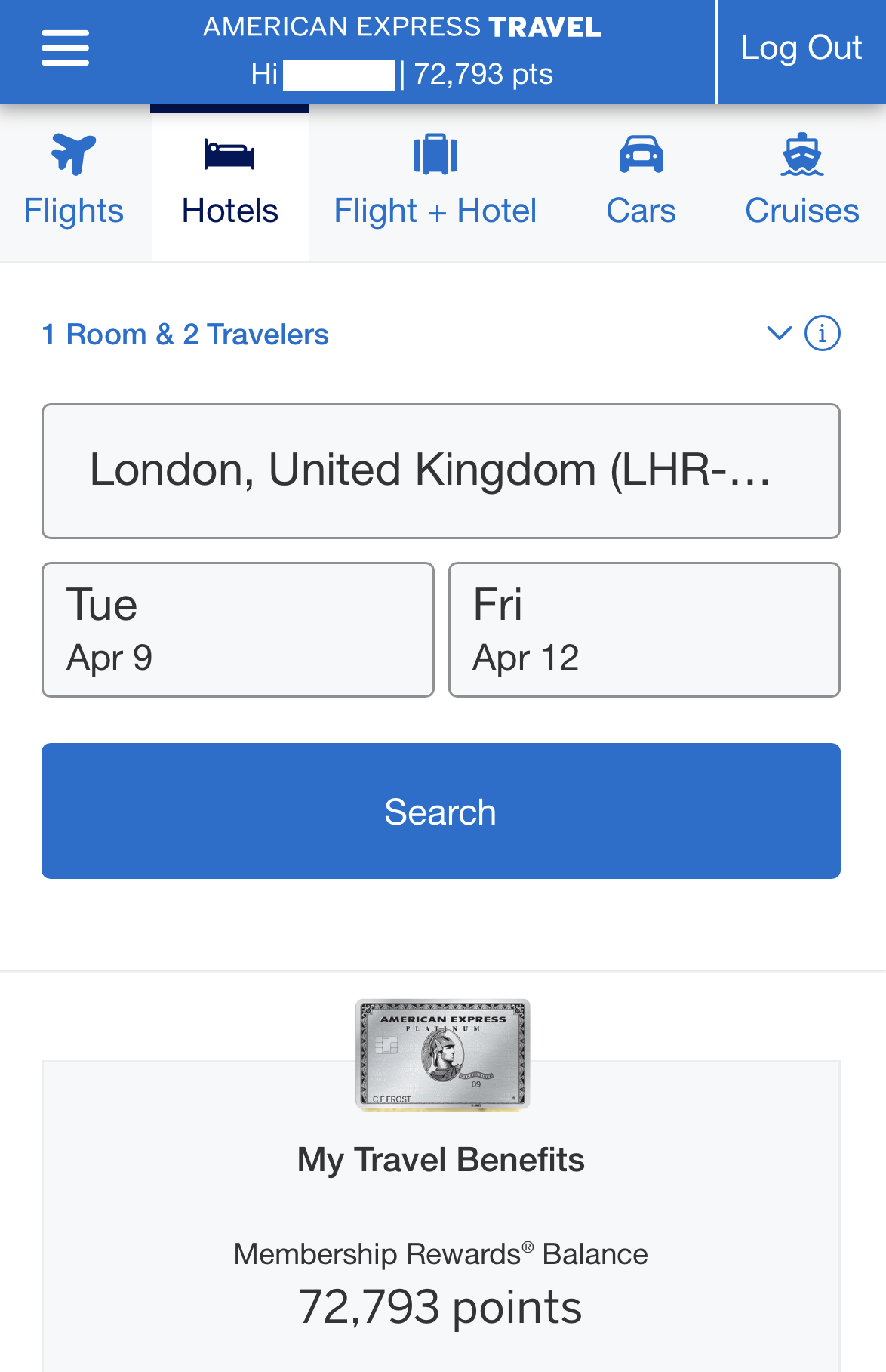Screenshot of American Express Travel App Interface

At the top of the app interface, there's a striking blue banner. On the left side of this banner, you'll find an icon with three horizontal lines, which typically indicates a menu. Prominently displayed at the top is the text "American Express Travel," with "Travel" in bold white letters.

Beneath this header, a greeting reads "Hi," followed by a username, which is redacted with a white rectangle. Adjacent to this, the user's reward points total, "72,793 points," is displayed. To the far right of this section, the option to "Log Out" is presented in white letters.

Below the banner are various category tabs for navigating the app: "Flights," "Hotels," "Flight + Hotel," "Cars," and "Cruises." The "Hotels" tab is currently highlighted. In the section beneath, the app specifies "1 room and 2 travelers" in blue text. There is also a dropdown box and an information icon situated to the right.

Further down, there are input fields for travel details. The destination field is pre-filled with "London, United Kingdom," along with its airport code. Two date fields lie below, designated for "Depart" and "Return" dates.

The search function is highlighted by a large blue bar stating "Search" in white letters. Beneath the search bar, there's a thumbnail image of an American Express card, centered under which are the words "My Travel Benefits."

At the bottom section of the app, the "Membership Rewards Balance" displays the same reward points total, "72,793 points."